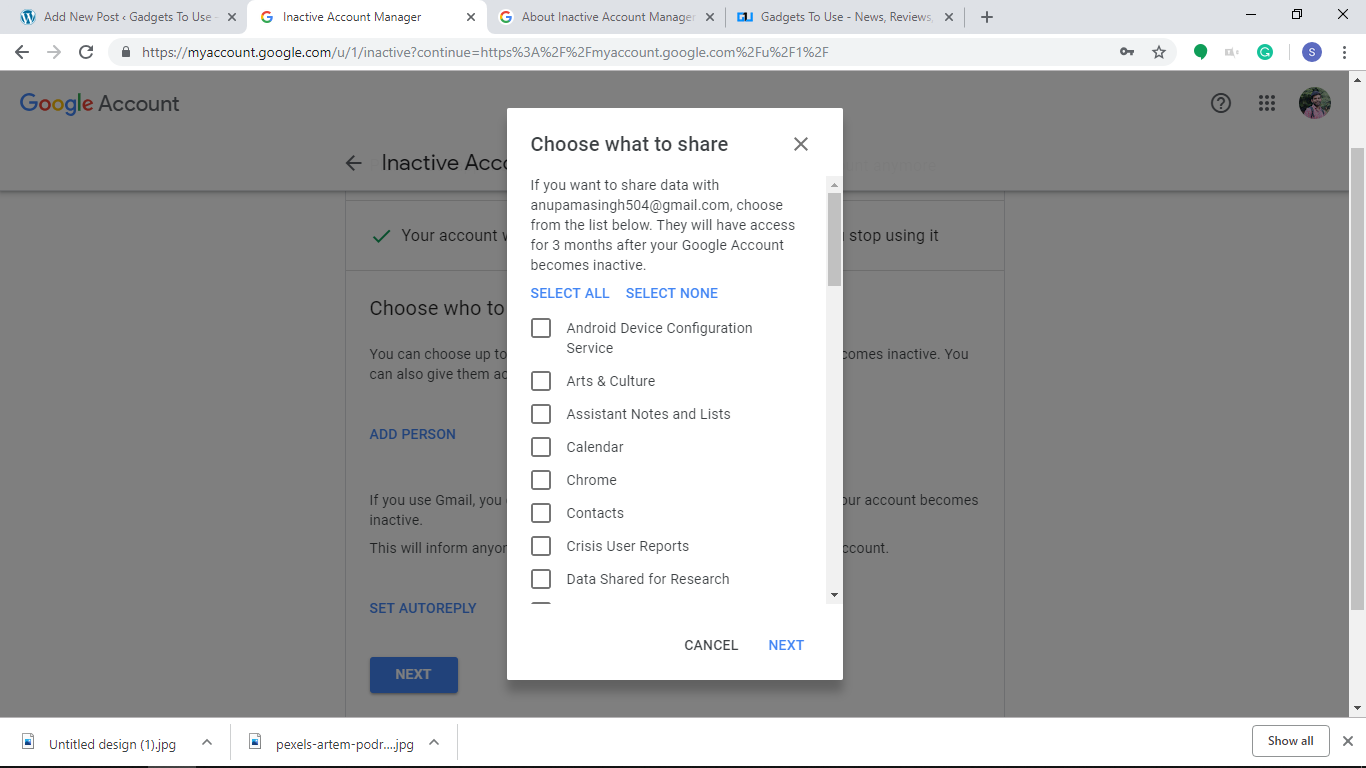The screenshot showcases a user interface for managing an inactive Google Account within a website. At the top of the interface, a gray bar with black text displays the option "Add New Post." Below this are tabs, with the second tab titled "Inactive Account Manager" highlighted in white, indicating it is the active selection. The other tabs include "Active Account" and "Gadgets to Use," rendered in gray with black text.

The left side of the interface features a vertical gray bar with minimized window controls, including minimize, windowed view, and exit buttons.

Below this, the layout includes a white background with various navigational elements. A black arrow pointing to the left is followed by a series of buttons: a gray "Back" button, a black "Refresh" button, and an address bar displaying the current URL. Beside the address bar are icons including a key, a star, a question mark, and a speech bubble, each with specific functionalities. The user's Google Account avatar, represented as a white 'S' on a blue background, appears next to these icons.

At the top left, in the Google colors, the "Google Account" title stands out against a gray background. On the right side, additional icons include a question mark within a circle, a 3x3 grid of dots, and the user's profile picture.

The main content area displays a pop-up for managing "Interactive Account" settings. The pop-up, on a white background, prompts the user to "Choose What to Share," with a gray 'X' button to close the prompt on the right side. Beneath the prompt, gray text informs the user that if they want to share data with someone's email address at gmail.com, they should choose from the provided list. This shared access will last for three months after the user's account becomes inactive.

Options listed for sharing data include:
- Android Device
- Google Arts & Culture
- Assistant Notes
- Calendar
- Chrome
- Contacts
- Google Play Preferences
- User Activity Reports

At the bottom of the pop-up, there are two buttons: "Cancel" and "Next," both in black text.